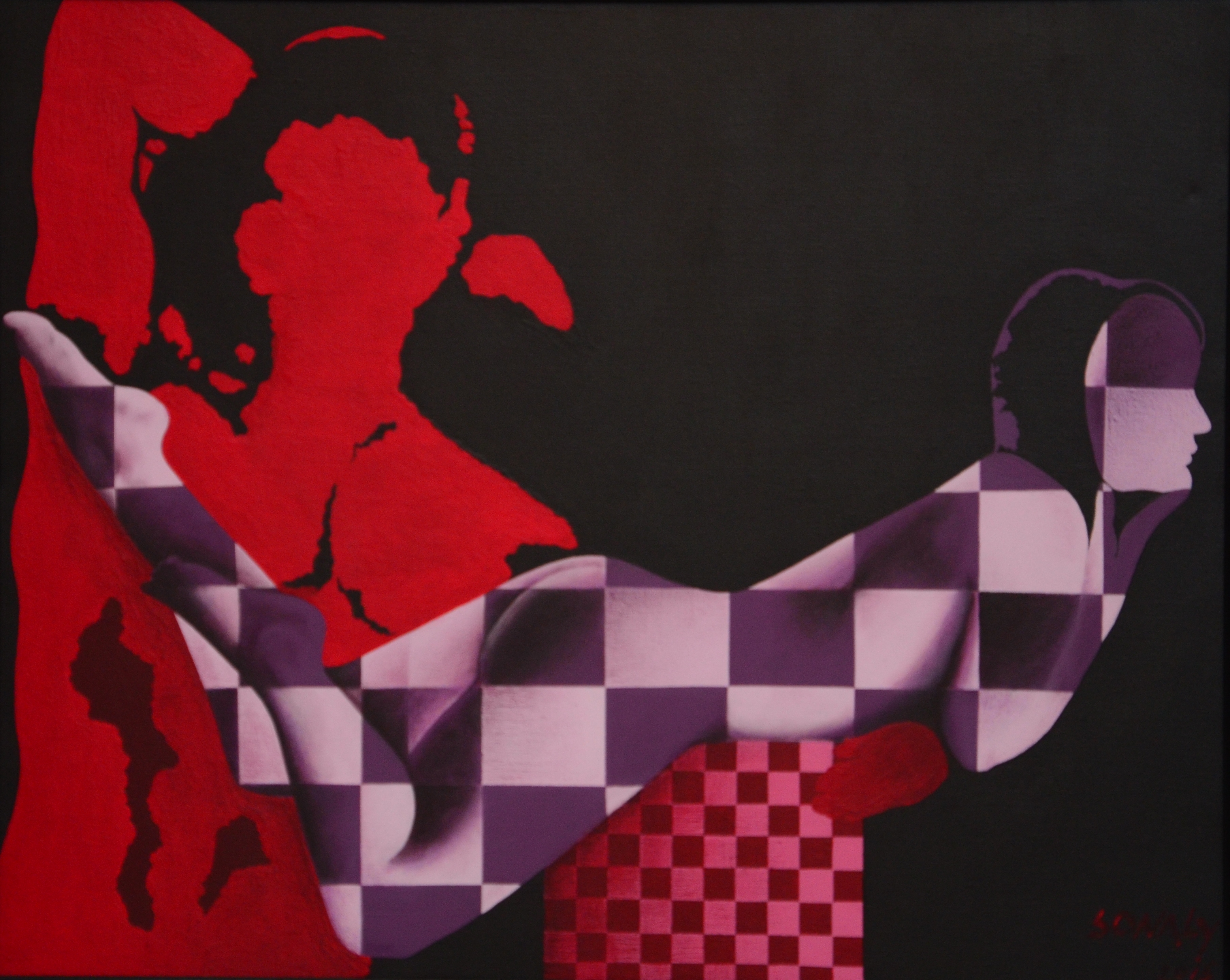A detailed digital collage features a textured black background. On the left side, an abstract red silhouette of a figure, possibly a male or female, is shown from the waist up, with longish hair and the right arm raised, elbow bent, and forearm with hand positioned behind the head. The figure's head touches the top of the frame while the waist is at the bottom. In the center bottom of the image, there is a small square checkerboard in pink and red. Across the middle of the composition, a second silhouette of a woman stretches horizontally, lying on her belly with bent legs and feet kicked up. Her hands are tucked under her chin in a relaxed pose. This central silhouette is rendered in a gray and dark purple checkerboard pattern, contrasting vividly with the background and other elements.